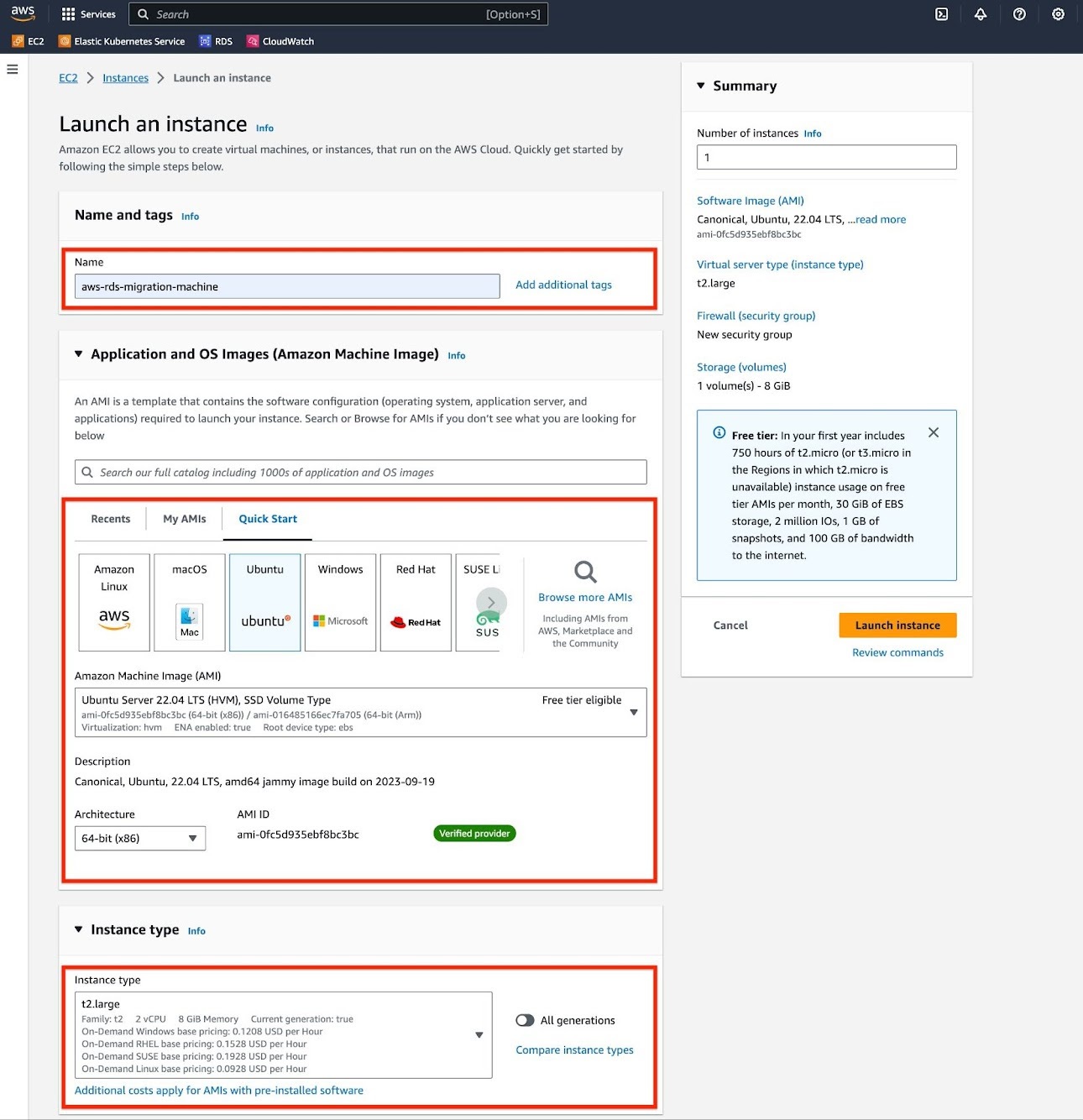This image depicts a web interface against a black background, prominently featuring Amazon Web Services (AWS) elements. In the upper left corner, the AWS acronym and Amazon logo are displayed, indicating that the interface is related to Amazon Web Services.

Below the logo, a navigation bar includes a 3x3 white grid icon, followed by the word "Services." To the right of the navigation bar, there is a gray search bar, and further right, icons for a tab menu, notification bell, help circle, and settings gear are visible.

On the left-hand side of the interface, the services EC2 (Elastic Compute Cloud), RDS (Relational Database Service), and CloudWatch are listed in a vertical white column. This column also features an icon with three black horizontal bars in the upper left.

Within the main interface, an introductory section for EC2 Instances is present. The blue underlined text reads "EC2 Instance," and below it, in black text, "Launch Instance" is written. Additional text explains that EC2 allows the creation of virtual machines or instances on the AWS cloud and provides a quick start guide for new users.

The form below has multiple input fields including a red-circled section for naming the instance. Additional fields and red-circled annotations discuss recent supply AMIs and quick start templates focusing on macOS, Ubuntu, Windows, and Red Hat operating systems.

A segment of the form focuses on configuring instance types and includes a brief summary section on the right. At the bottom of the page, summary details are provided to finalize the setup, though some text is partially obstructed or unclear in the image. 

Overall, the image captures a detailed section of the AWS management console, specifically tailored for launching and configuring EC2 Instances.